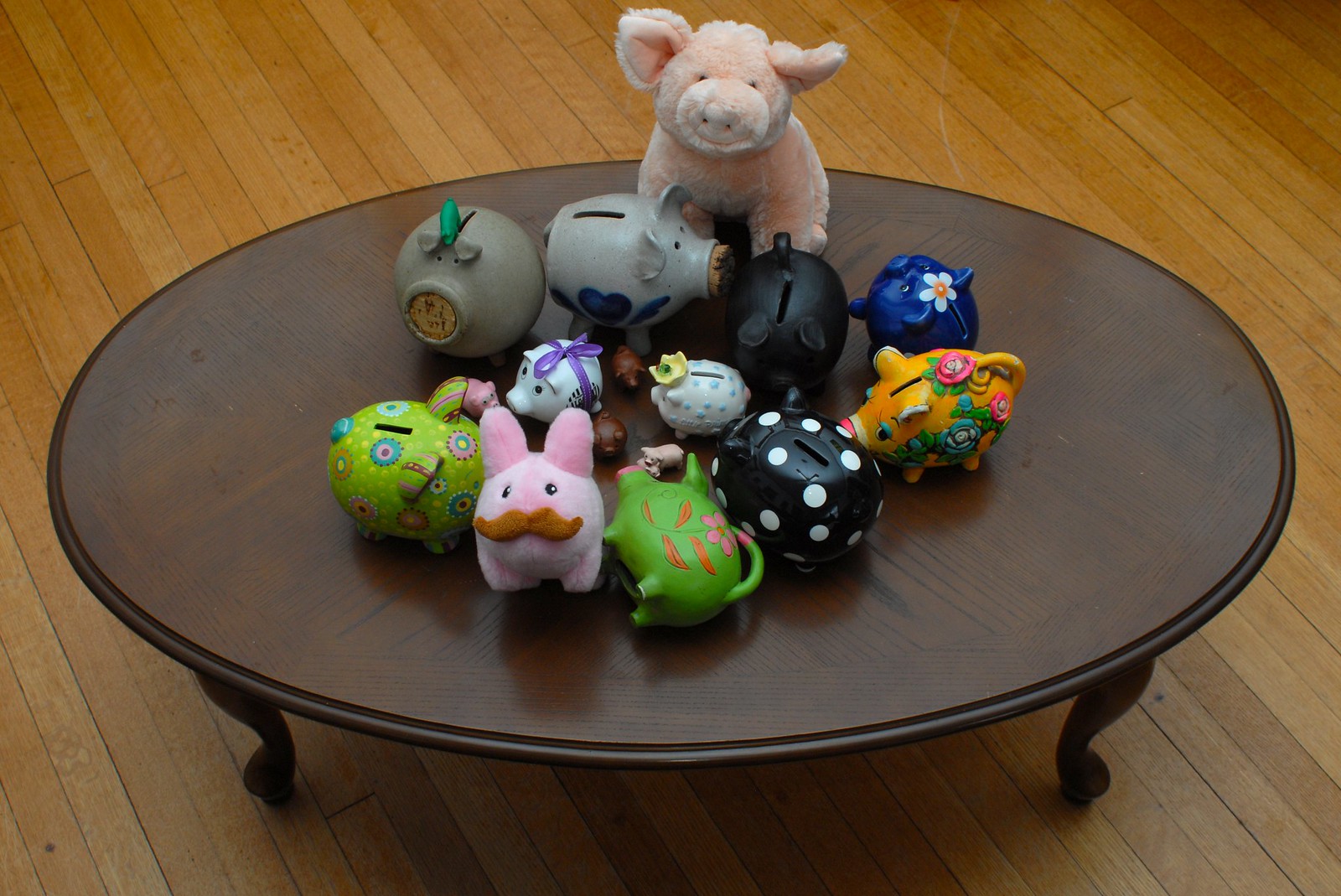The image features a round coffee table made of dark-stained wood, standing low to the ground at approximately 10 inches high, with short legs. The perspective of the photo is an overhead shot, giving a bird’s-eye view. The table sits on a wooden floor comprised of thin planks. The surface of the table is adorned with an eclectic collection of pig-themed items. These include stuffed pigs and various piggy banks of differing colors and designs. The centerpiece is a notably larger, fuzzy stuffed pig of an orangish-pink hue. Surrounding it are multiple small piggy banks: two gray ones, a black pig with white polka dots, a red pig with a white daisy on its head, an orange pig decorated with pink flowers and greenery, and several pink piggy banks with various designs. Among the collection, there's also a yellow pig with floral patterns and a tiny pink pig with a tan mustache. Additionally, two miniature pigs are nestled in the middle of the table, and a unique pig lying down, painted green. The lighting in the photo is dim, casting low light across the scene, which highlights the dark tones of the table and the colorful array of pig figures.